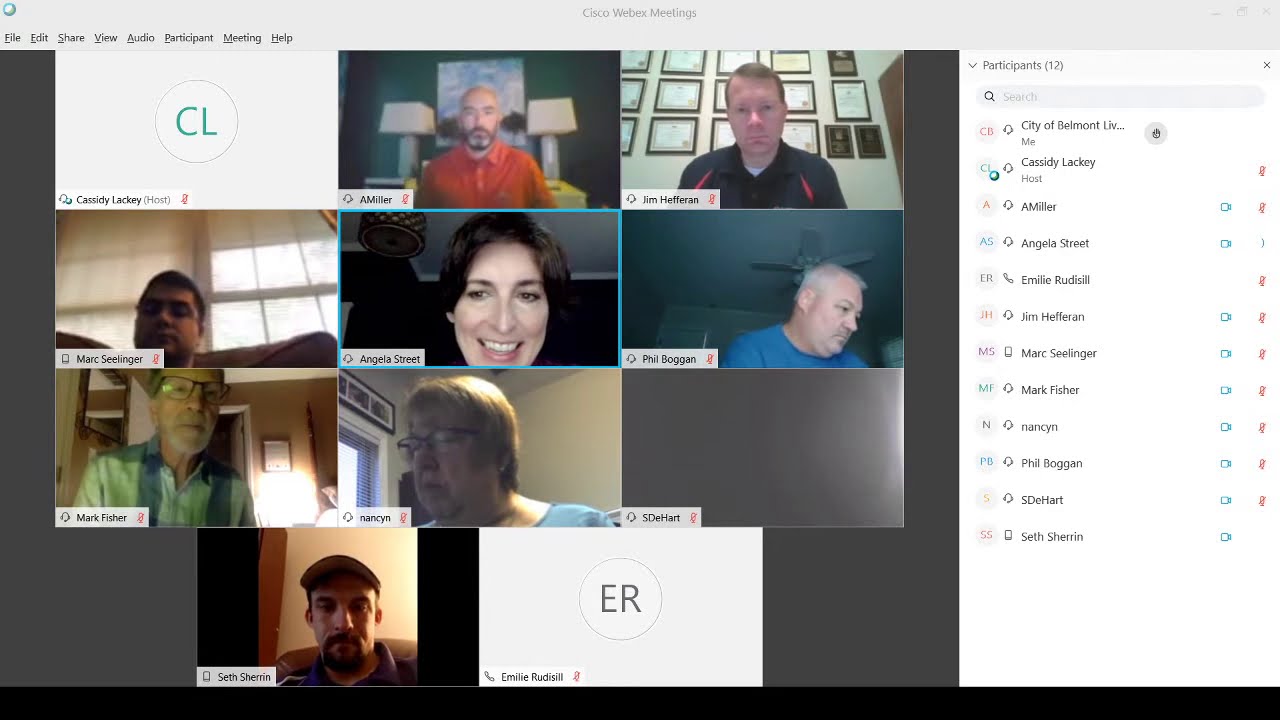This screenshot depicts an ongoing Cisco WebEx meeting, prominently labeled at the top center. The screen is divided into multiple sections, with the upper left corner featuring commands such as file, edit, share, view, audio, participant, meeting, and help. The right-hand side showcases a detailed participant list, revealing a total of 12 attendees. 

The central section of the screen mimics the iconic Brady Bunch format, displaying a grid of 11 windows over three rows of three and one row of two. Nine windows display participants, including a bald man with a beard in a red polo shirt, a man in a black shirt, and two men flanking a woman in the middle row. The next row shows an older man, a middle-aged woman, and an empty gray screen with just a name displayed. The bottom row includes a man wearing a cap with a goatee, a younger man in his 30s, and another window with only the initials "ER."

Two windows feature only initials in a circle: "CL" in the top left corner and "ER" in the bottom. The participants range from middle-aged to elderly, with control options for muting and camera settings visible to the moderator on the right-hand side. This detailed layout and participant configuration emphasize the virtual meeting's organized structure.